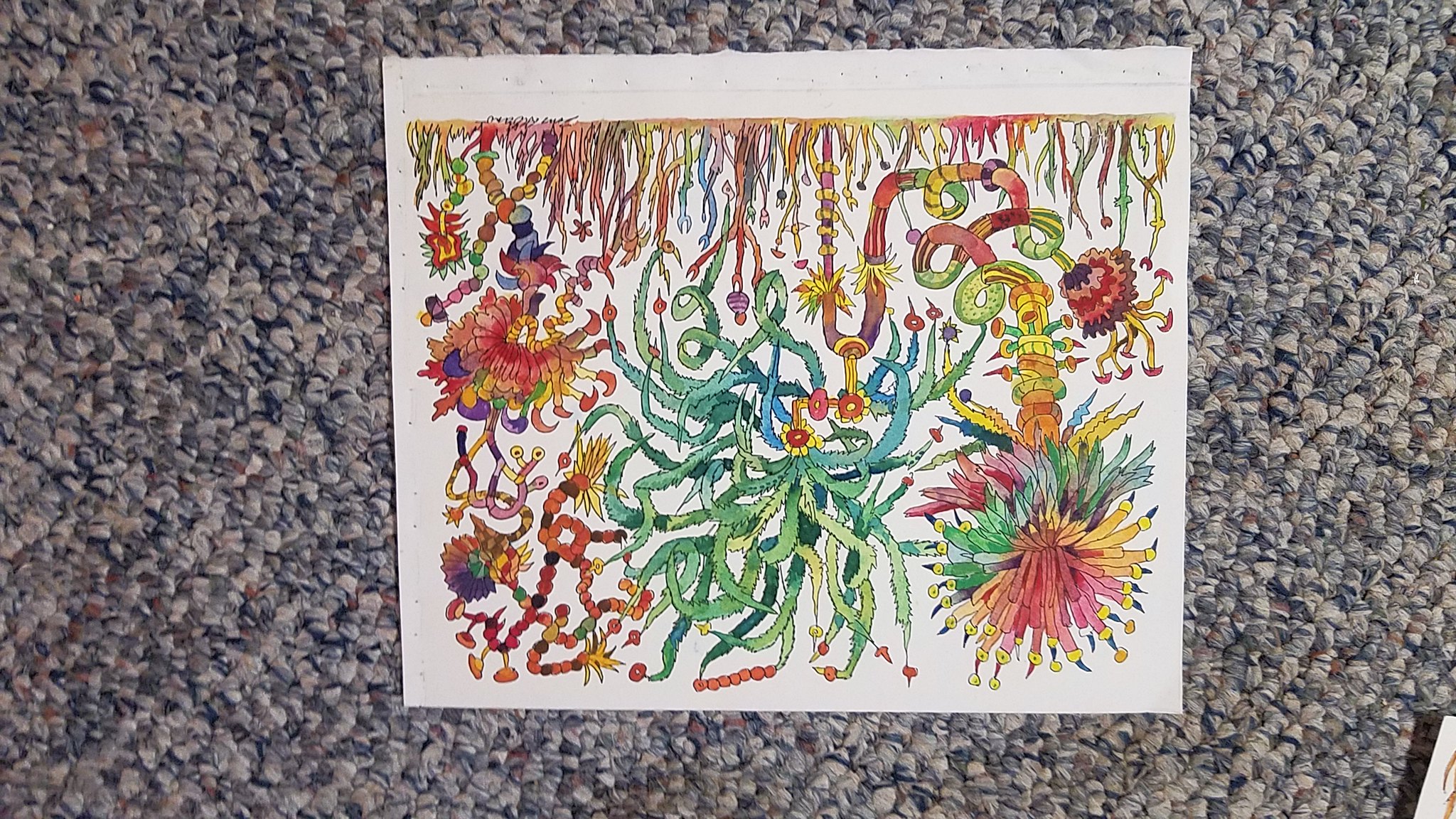This is an intricately detailed, psychedelic drawing done on a white piece of paper with jagged edges, suggesting it was ripped from a book. The artwork, created with either watercolors or colored markers, lies on a textured Berber carpet with blue, white, gray, and black flecks. Dominating the center is a vibrant green plant resembling seaweed, with numerous skinny leaves sprawling in every direction. Surrounding it are multicolored elements, including rainbow-hued starburst flowers and interwoven leaves in oranges, reds, greens, blues, and yellows. The top of the image features fringe-like tinsel strands or roots in various colors. The entire scene evokes an otherworldly, almost Dr. Seussian landscape and may be oriented upside down.